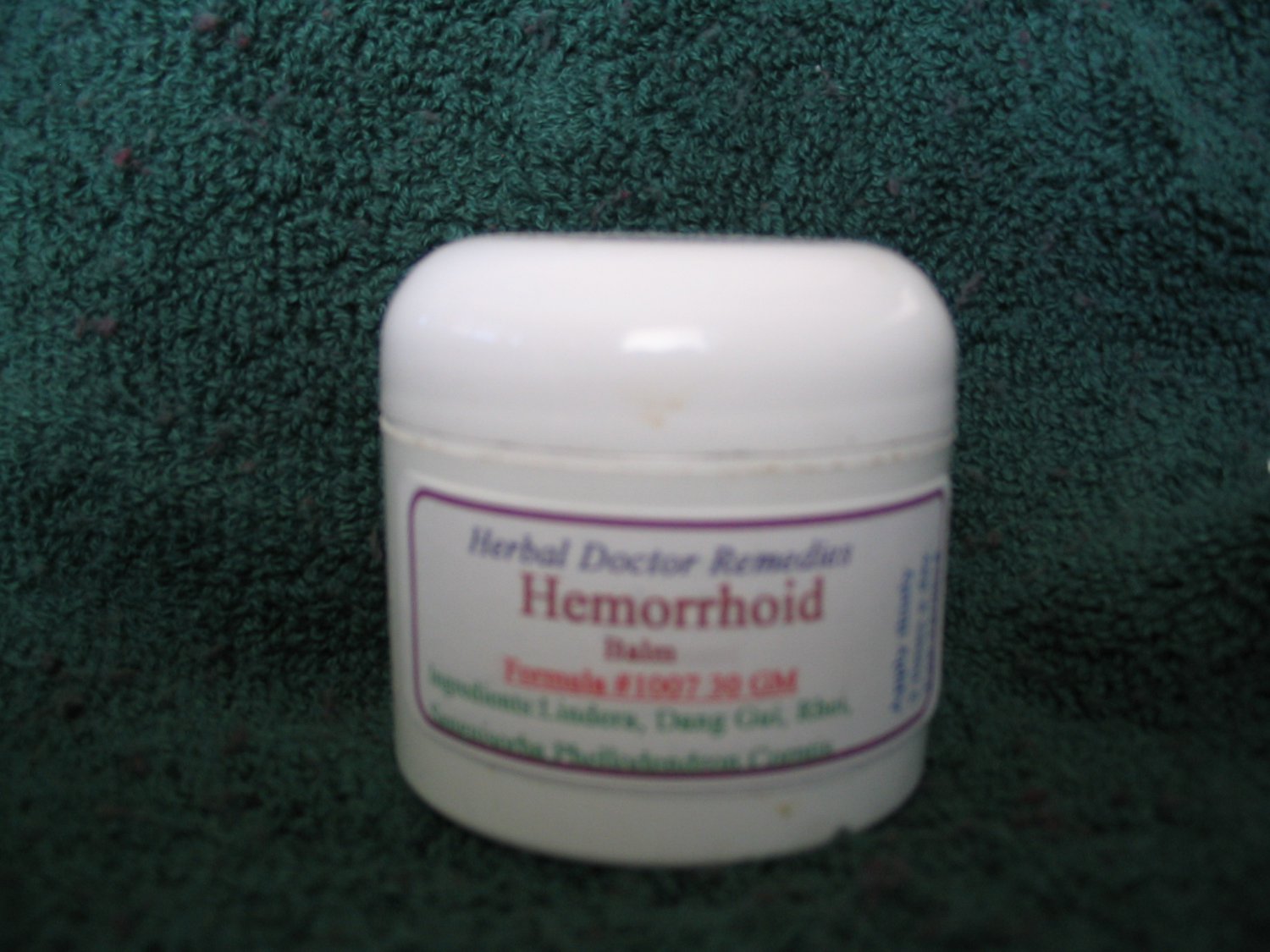In this color photograph, set in landscape orientation, the central subject is a round, short plastic container of hemorrhoid balm. The container features a screw-on, dome-shaped lid that is flat on top. It rests on what appears to be a dark green fabric, likely a towel, blanket, or sweater, providing a soft, textured background. The white label on the container, bordered by a dark purple rule, prominently displays the text "Herbal Doctor Remedies" in black italic at the top, followed by the word "Hemorrhoid" in red, and "Balm" in smaller red letters underneath. A formula number is also visible in red text below these words, with additional product attributes listed in green type underneath. The label includes more text along its right side, likely listing the ingredients, though this text is somewhat blurred and difficult to read. The rich color palette of the image features shades of green, brown, purple, red, dark red, and blue, accentuating the product's details despite the slight out-of-focus effect of the photograph. The setting suggests a home environment, captured in a style that blends photographic realism with representationalism and product photography.